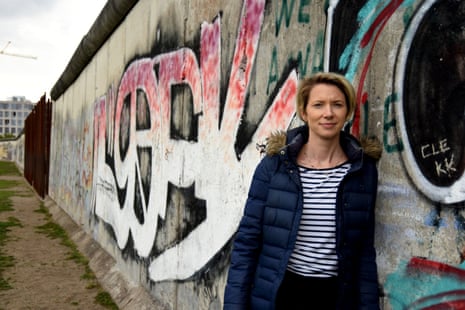The image is a photograph of a middle-aged woman standing in front of an extensive, concrete wall covered in varied graffiti, including both words and pictures. The graffiti features the word "CLEKK" and an array of colors like blue, green, red, white, and black. Some of the graffiti also has white letters with reddish-orange tops. The wall, which extends far into the background, suggests a sense of depth and a cold, dreary atmosphere. The ground around the wall has sparse grass. The woman, who has short, cropped blonde hair, appears to be leaning against the wall. She is dressed in a navy blue parka with a fur-trimmed hood over an open navy and white striped t-shirt, and black pants. She looks directly at the camera with a slight smile. In the left part of the background, a portion of a building can be seen near a sidewalk with patches of green grass.